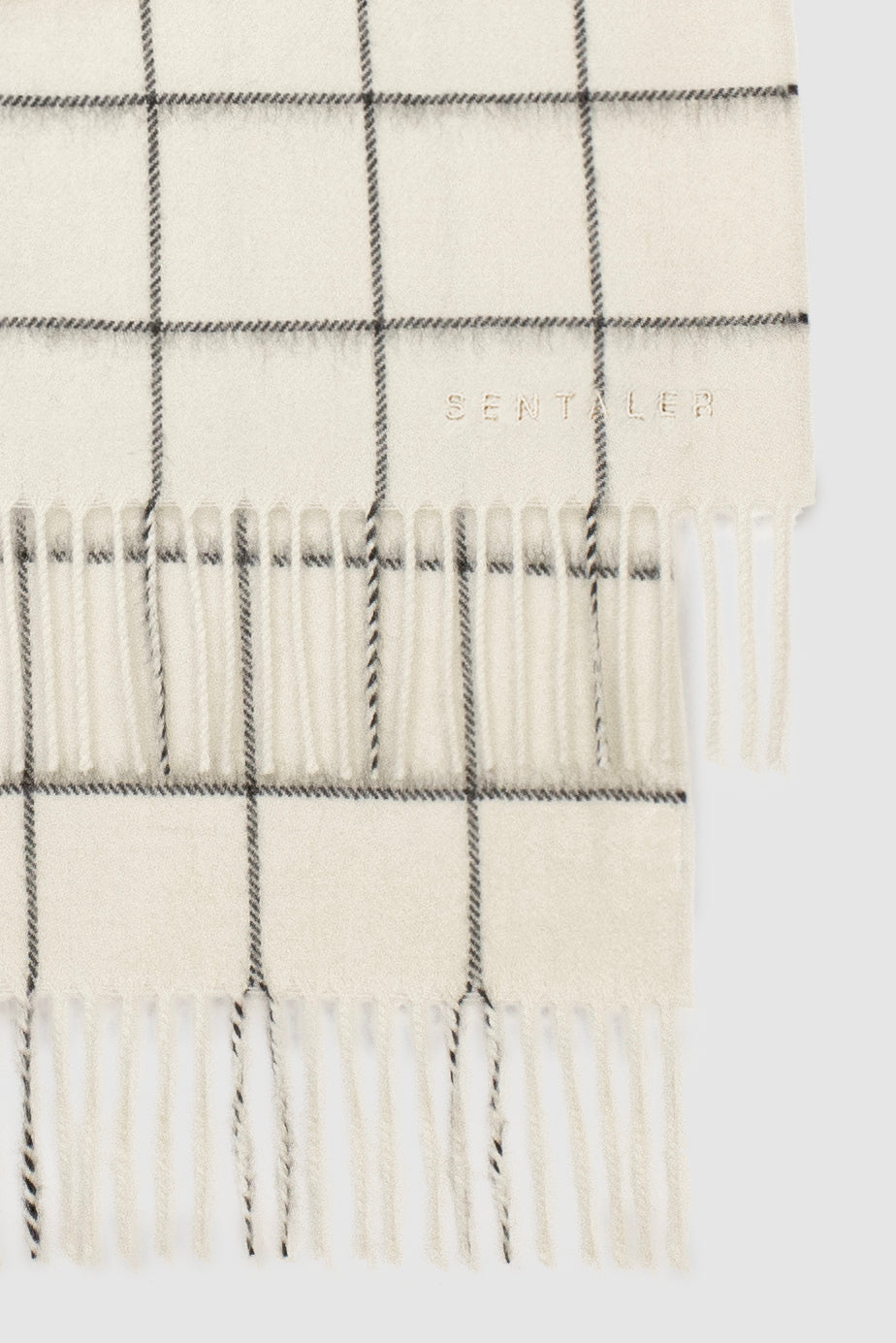This close-up photograph captures a detailed view of a fabric, likely a scarf, with a distinctive black grid pattern against an off-white or cream-colored background. The material exhibits two layers laid on top of each other, each adorned with evenly spaced, braided fibers extending from the ends, creating a tasseled effect. The pattern, resembling a checkered or kitchen-like design, seamlessly continues through these offshoots, enhancing the overall aesthetic. Amidst the intricate design, a logo reading "SENTALER" is embroidered in the corner, adding a touch of branding to the sophisticated fabric. The combined elements of the twisted ropes, brown and white threads, and the flowing tassels suggest the material would exhibit a captivating movement if caught in the wind, enhancing its elegant and unique design.